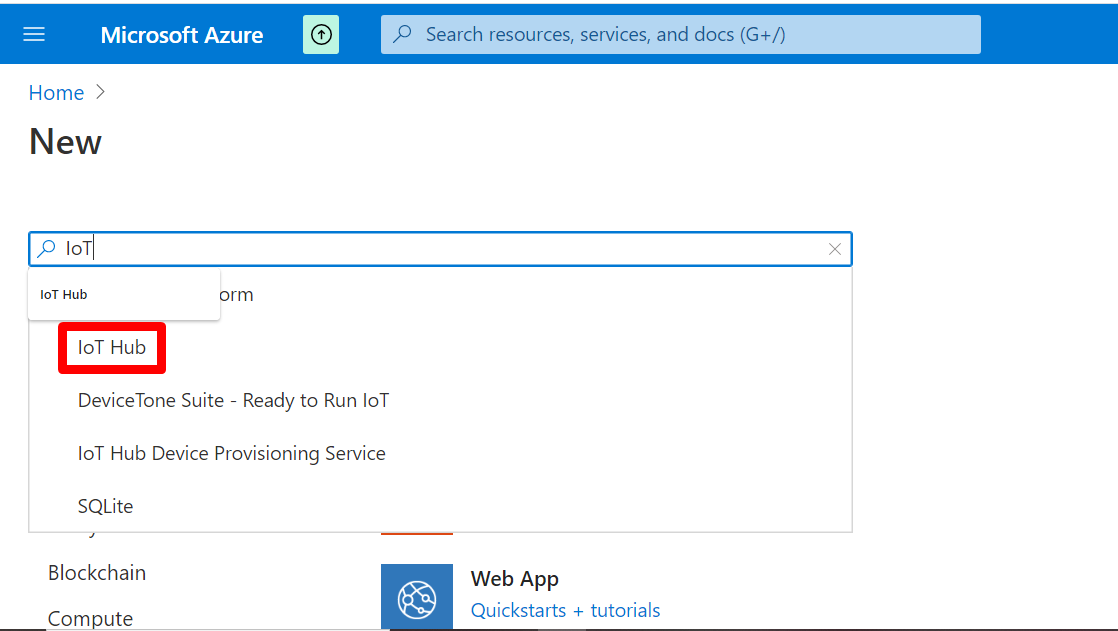This image is a vertically-oriented screenshot, most likely captured from a laptop or computer, displaying a website without clearly defined borders. At the top of the screen, there is a horizontal blue header. On the left side of this header sits a white hamburger menu icon, followed by the text "Microsoft Azure" in white font. Next to the text is a small green box containing a black circle with an upward-pointing arrow inside. To the right of these elements is a long, rectangular, light blue search bar with a magnifying glass icon on the left; this search bar contains the placeholder text, "Search resources, services, and docs," with the term "Google Plus" highlighted.

Directly below, there is a home button depicted in blue and a header with the word "New" in black font. Further down, there is another blue search bar, this one containing the partially typed text "L-O" followed by a capital "T" with a cursor flashing next to it, indicating an active search query.

The suggestion "lot hub" appears beneath this search bar as a clickable option. Below the suggested search, "lot hub" is displayed again but this time inside a long, rectangular red border, presumably highlighting it as the correct search item to select.